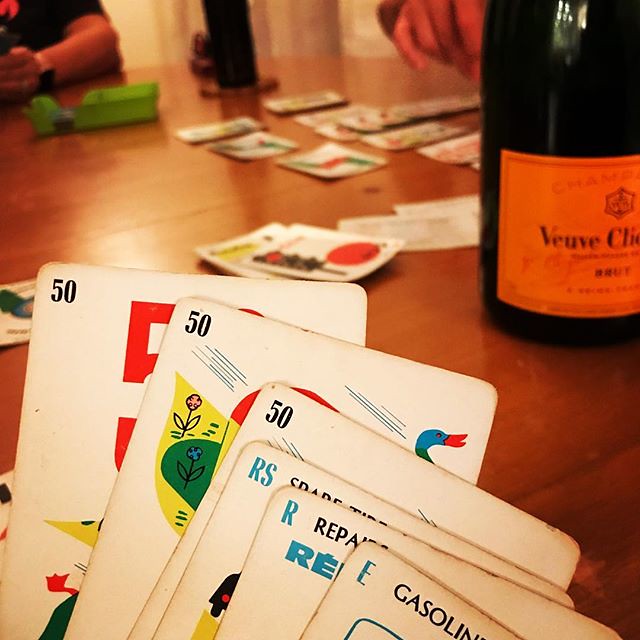A person is engaged in a card game, and the perspective is as if you were holding the hand of cards yourself. You can see six cards in total, although the player's hand is not visible. The cards shown include three with the number 50, and three others labeled RS, R, and E. The deck appears to be well-used, with browning edges adding to their vintage feel. The number 50 cards are marked in dark black at the top left corner, and only this portion of each card is visible. 

The second card in the array features intricate artwork, depicting a duck and a vibrant field with an orange flower, a blue flower, all set against a yellow background with a green patch near the blue flower. 

On the table below, cards are laid out in a pattern suggestive of a game like gin rummy. A bottle of Veuve Clicquot champagne with its distinctive orange label is prominently placed, though only its base is visible before it starts to taper. Behind the bottle, a hand is poised to pick up some cards. To the right, another person’s arm is visible, adorned with a gold watch with a black face. In front of this person, there appears to be a card deck dealt onto a green surface, possibly indicating the presence of a dealer.

This rich scene captures the essence of a vintage card game setting, filled with details and vibrant elements.